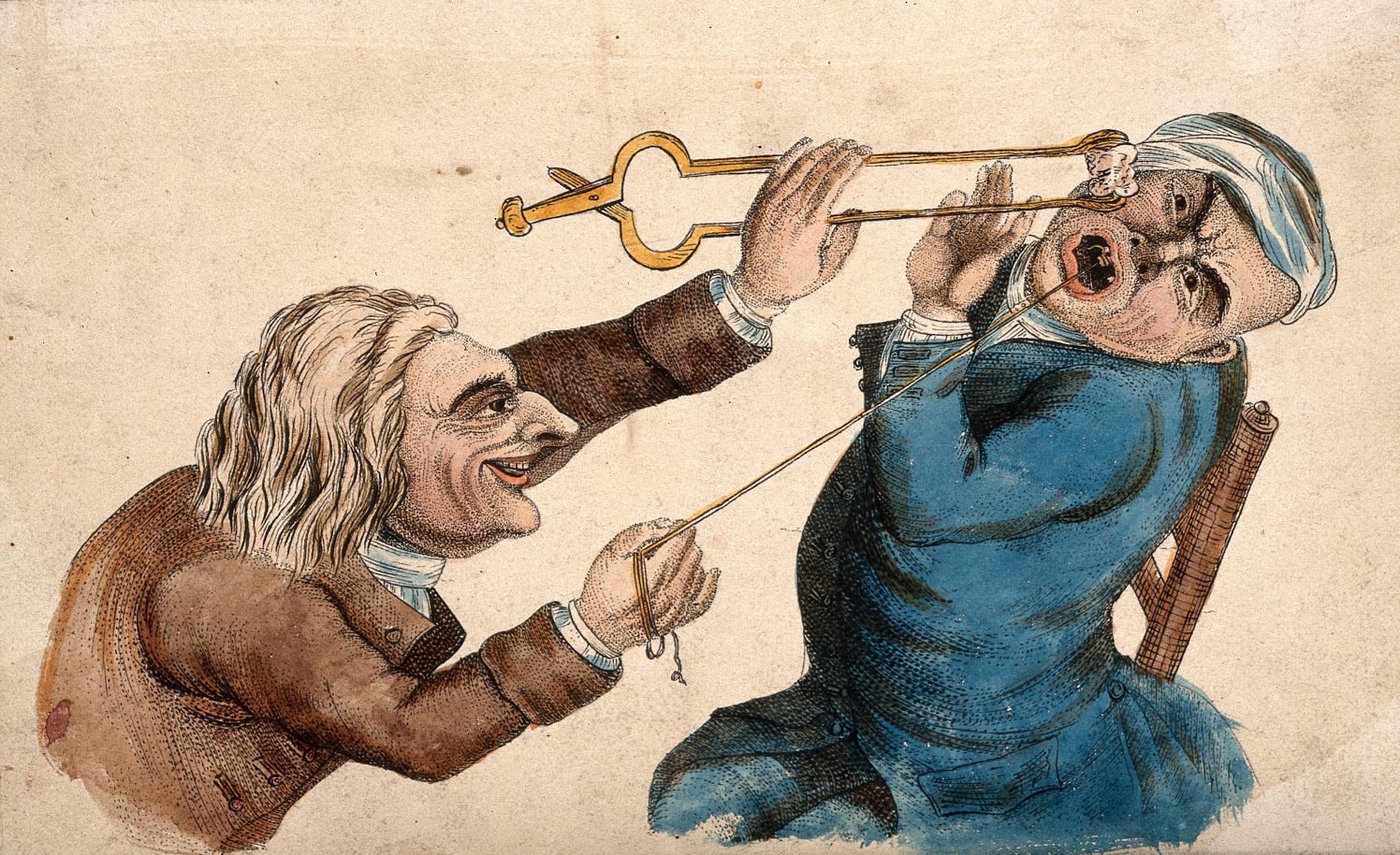This detailed painting depicts an archaic scene of a tooth extraction. Set against a mainly beige background with subtle black speckles, it portrays a dramatic interaction between two characters. On the left is a white man clad in a brown jacket, characterized by his long, blonde hair (depicted as gray in some interpretations), a pronounced long nose, and a long chin. With a sinister yet strangely friendly smile, he holds a piece of string in his right hand, attached to the tooth of the other person. His left hand wields a pair of forceps, possibly holding cotton or another white material.

The person on the right, trapped in the agony of the moment, wears a white headband and a blue jacket. His head is thrown back, his arm is raised, and he sits in a chair, clearly wincing in pain from the tooth extraction. The overall mood captured in this illustration resembles an antiquated textbook visual, emphasizing the crude methods of dental practices from the past.